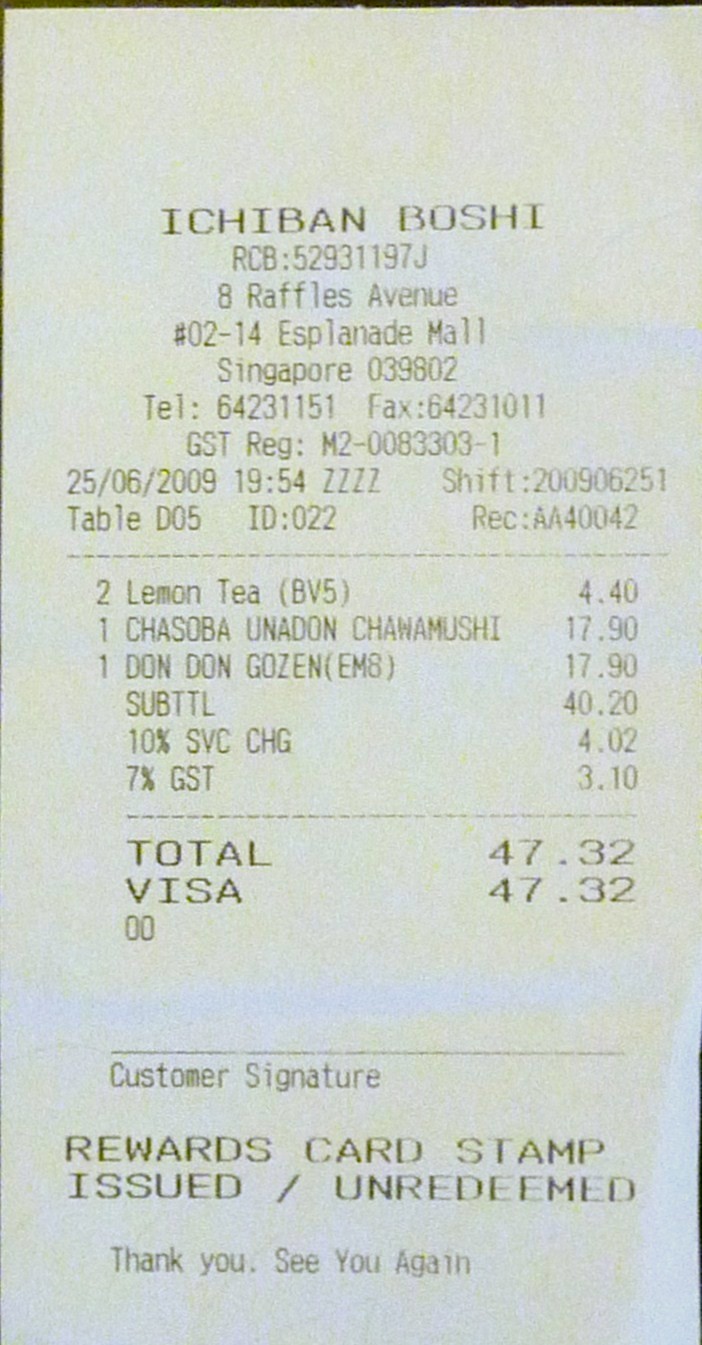A photograph or scan of a detailed restaurant receipt from Ichiban Boshi, located at 8 Raffles Avenue, #02-14 Esplanade Mall, Singapore. The receipt is dated June 25, 2009, at 7:54 PM. It provides a detailed breakdown of the order, including two Lemon Teas for $4.40, one Cha Soba Unadon Chanamushi for $17.90, and one Don for $17.90. The subtotal for the meal is $40.20, with an additional 10% service charge amounting to $4.02 and a 7% GST (Goods and Services Tax) of $3.10. The total bill comes to $47.32, paid by Visa. There is a blank space for a customer signature and a note at the bottom stating "Rewards card stamp issued/unredeemed. Thank you, see you again." The receipt also contains various numbers used by the restaurant for tracking orders, including a shift number and a table number.